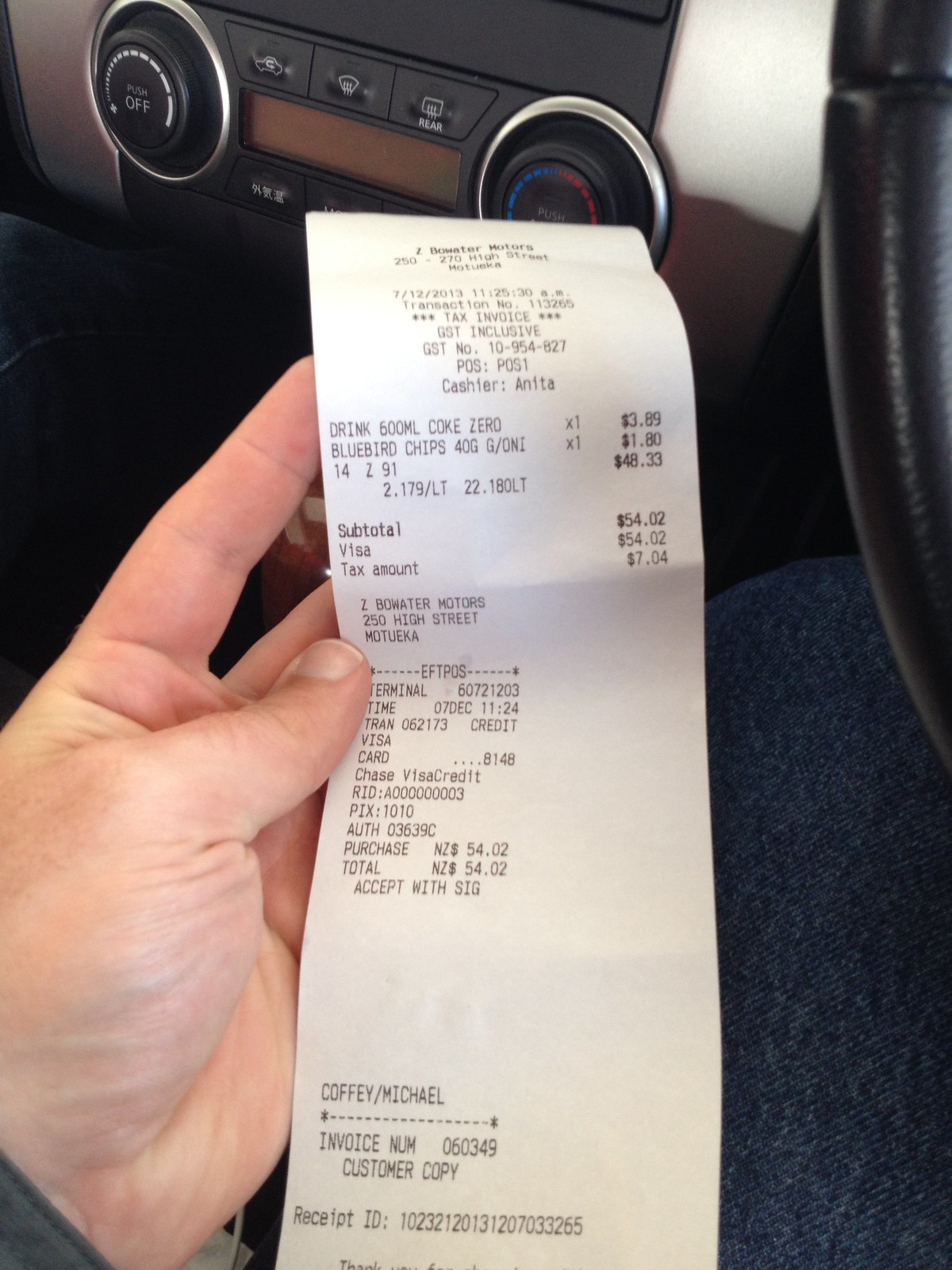In the photograph, a person is seated in their car, holding up a receipt in their left hand. The steering wheel is visible on the right-hand side of the image, suggesting that the car is from a country where driving is on the left side of the road. Additional details inside the car include HVAC control knobs and Asian lettering. The receipt is from Z Bowater Motors, located at 270 High Street, Motueka, New Zealand. The receipt, addressed to Michael Coffee, lists the purchase of a Coke Zero for $3.89, Bluebird chips (40 grams) for $1.80, and 14 liters of gasoline priced at $48.33, totaling $54.02 before tax. The tax amount is $7.04, and the purchase was completed using a Visa Chase credit card. The receipt also includes terminal information and card details.